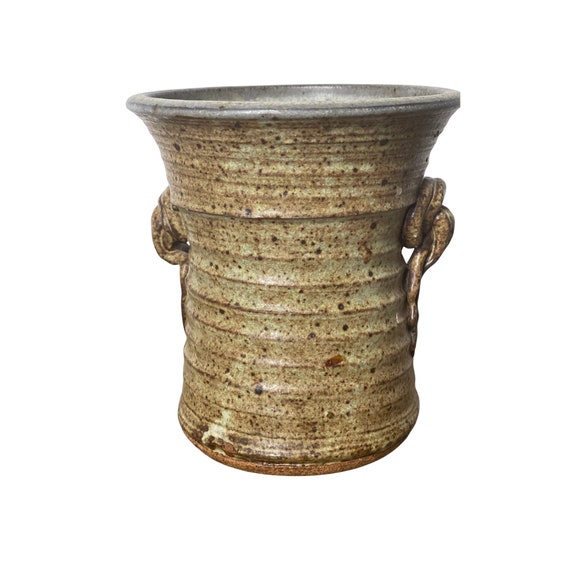This image showcases a photorealistic depiction of a very old-looking vase or ceramic water vessel, centrally positioned against a plain, flat white background. The vase has a generally cylindrical shape, ribbed horizontally with multiple lines encircling its body. The upper part of the vase features a flared opening that is more gray in color. The overall color of the vase is a light brown, speckled with much darker brown dots across its surface, giving it an unweathered, yet aged appearance. On either side of the vase, there are stylistic dark brown attachments that resemble rope-like handles, seemingly crafted from the same material as the vase itself. Despite its ancient design, the vase appears to be in remarkably good condition, possibly indicative of its historical significance as a water-carrying vessel.